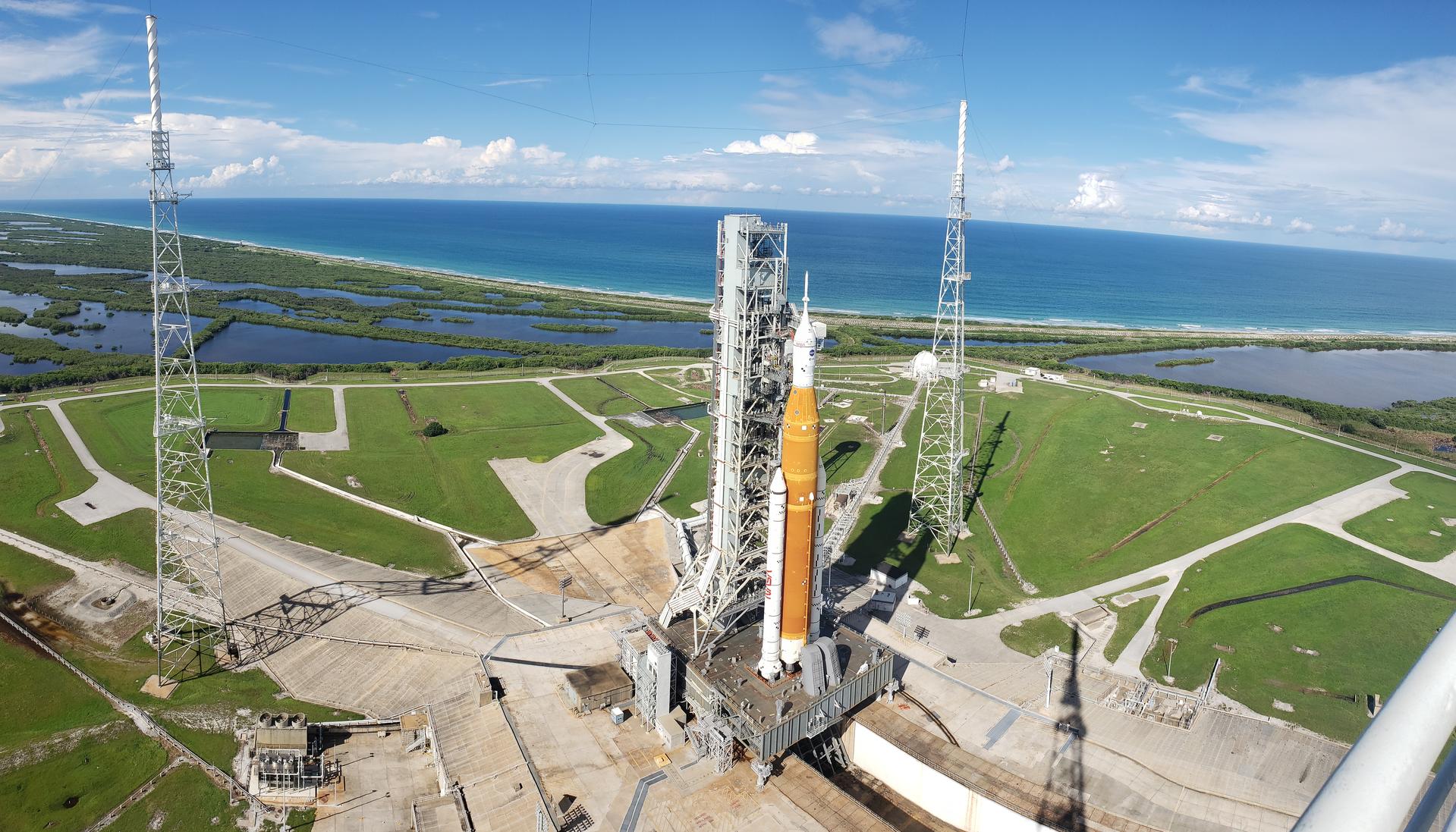The image depicts a detailed aerial view of a rocket launch site, likely NASA's, situated along a waterfront, presumably in Florida, with the blue ocean visible in the backdrop. The sky above is clear with wispy white clouds. The centerpiece is a large rocket positioned on a cement launch pad. The rocket is primarily orange-rust colored with white boosters on either side and a white capsule at the top. Flanking the launch pad are two tall, metal lattice towers equipped with large gantry cranes, which facilitate work on the rocket. The immediate surroundings of the launch pad feature a mix of concrete and paved areas extending in various directions, along with a designated trough for exhaust gasses during launch. The landscape also includes patches of green grass and marshy waters interspersed with green vegetation. There are small roads and pathways radiating out from the launch site, adding a sense of organized complexity to the scene.